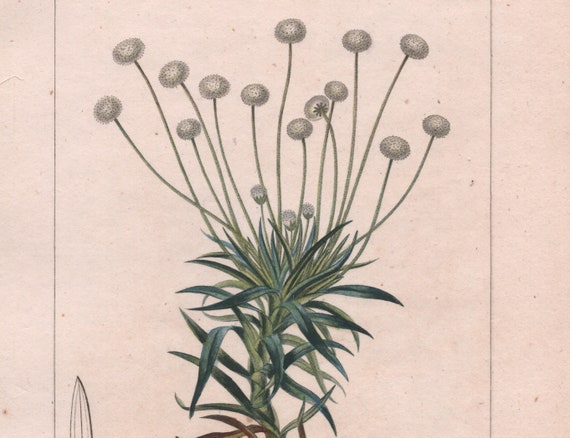This detailed illustration of a plant is reminiscent of vintage botanical drawings found in antique science books. The plant is depicted with a long central stem, from which numerous dark green, bushy leaves extend. Rising from the middle of the primary stem are multiple offshoots, each terminating in a fluffy, tufted cap that evokes the appearance of dandelions gone to seed. The background of the image is a faded pinkish beige, resembling old, aged paper and providing a stark contrast that accentuates the vivid green tones of the plant. The meticulous detailing of the illustration suggests it could be part of a detailed study or documentation in a research paper. An additional, slightly enigmatic element is present to the left of the plant, described as a jagged object that resembles a knife, though its inclusion and purpose remain unclear.